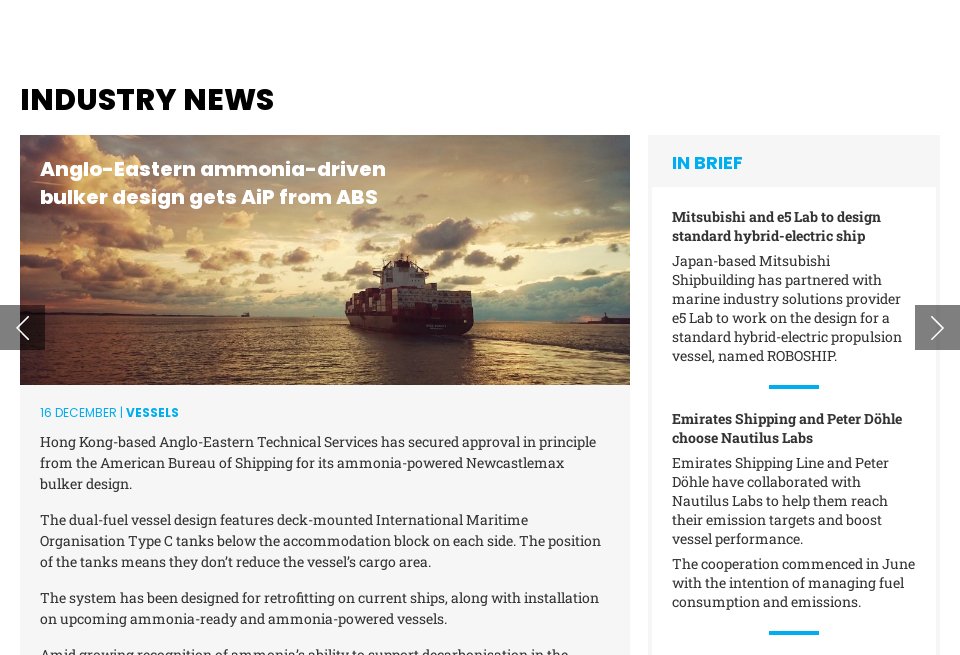In the image, we see a large ship navigating through gray waters under a sky that has a mixture of gray and white hues. In the top left corner of the image, the words "Industry News" are prominently displayed in black text. Directly beneath this, in white text, it reads, "Anglo Eastern ammonia-driven bulker design gets AIP from ABS," indicating a recent development in ship design.

At the bottom of the image, the date "16 December" is shown in blue text next to the word "Vessels." Beneath this, there are a few sentences written in black text that provide additional details about the aforementioned article.

On the right-hand side of the image, there is a section with a light gray background titled "In Brief" in blue text. Below this heading, another article is highlighted with the title, "Mitsubishi and E5 lab to design standard hybrid electric ship." The accompanying text explains that the Japanese-based Mitsubishi Shipbuilding has partnered with marine industry solutions provider E5 Lab to develop a standard hybrid electric propulsion vessel named Roboship.

Further down, another article is briefly mentioned: "Emirates shipping and Peter Dohle choose NAUTILUS labs,” accompanied by some informational text. Additionally, each article on the right-hand side of the image has a small light blue bar at the bottom, providing a subtle touch of color to the layout.